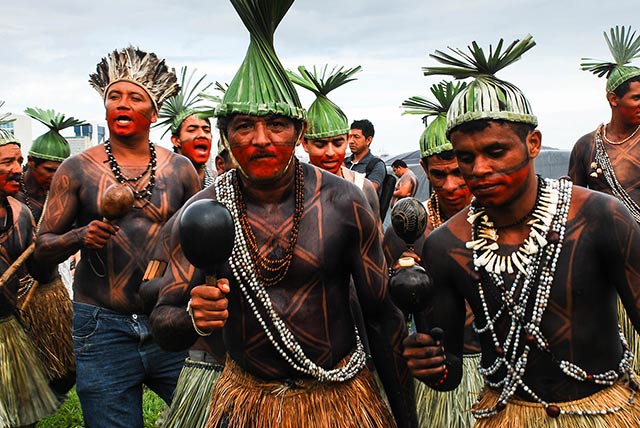The image depicts a group of aboriginal Mesoamerican men participating in a ceremonial dance, adorned in traditional attire. They have slightly brown skin and are shirtless, their torsos intricately painted with dark geometric patterns. The men wear distinctive hats made of twisted reeds or palm-leaf fronds, varying in style from skullcaps with topknots to cone-shaped and feathered headdresses. Their faces are strikingly painted, with the bottom half in red and additional black markings on some individuals.

Each man holds a black gourd shaker rattle in his right hand, and many of them are dressed in either green or orange grass skirts. They are also adorned with necklaces made of white and gray beads, with one man sporting a necklace featuring large teeth. In the background, a couple of men not in ceremonial garb stand by, observing the dancers.